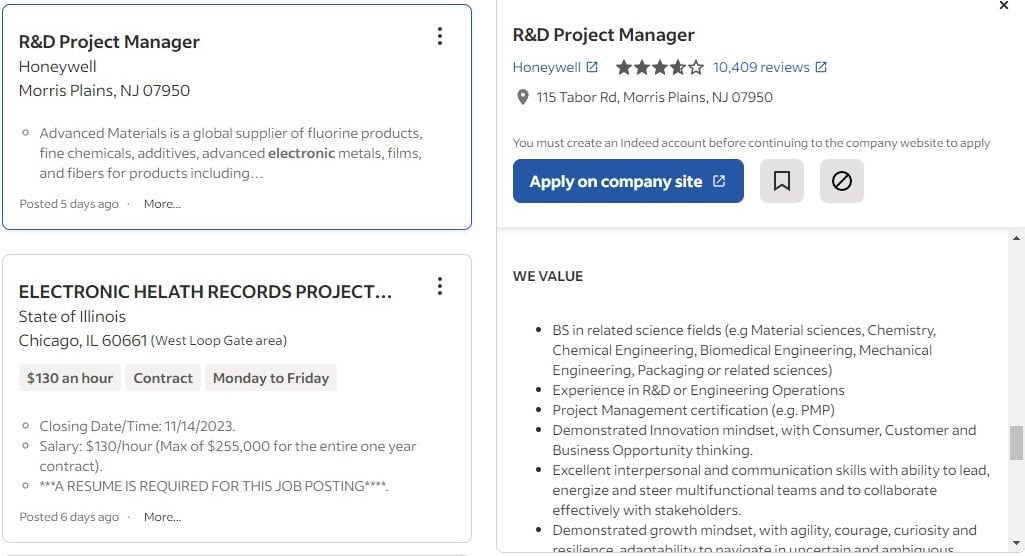This screenshot, taken from a web page, showcases four job advertisement boxes within a cropped view that excludes the web browser interface and page titles. A visible scroll bar is present on the right-hand side of the image, indicating additional content that can be viewed by scrolling. 

1. **Top Box**: The first advertisement is for a Research and Development Project Manager position at Honeywell. This box provides a brief job description and prompts the user to click for more detailed information about the role.

2. **Second Box**: This box advertises a position for an Electronic Health Records project. Notably, the word "health" is misspelled as "helath." The job listing includes information about the hourly rate, contract details, and the working schedule, which is Monday to Friday.

3. **Third Box**: Another Research and Project Manager role is detailed here. This box features a hyperlink for applicants to apply through the company's website. A list follows that highlights the company's valued qualifications and attributes, such as having a Bachelor's of Science in a related field.

Each box succinctly presents key job details, although some minor errors and abbreviations are present, like the misspelling in the second listing.